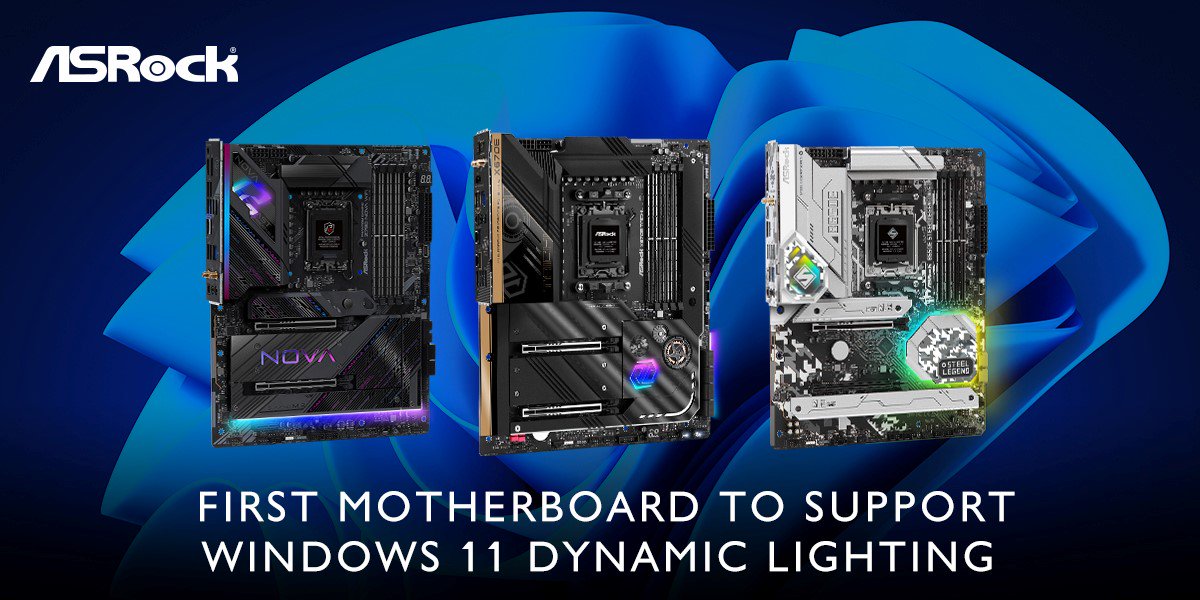This image is an advertisement for ASRock, showcasing the first motherboard to support Windows 11 Dynamic Lighting. Dominating the center are three square computer components: the two on the left are predominantly black, while the rightmost one is black with noticeable white details. These components feature rainbow lighting accents, particularly prominent on the third item. The background is an artistic, dark blue setting with a luminous, floral-like design adding depth. In white text at the bottom, the ad highlights, "First Motherboard to Support Windows 11 Dynamic Lighting." The ASRock branding is marked clearly in the upper left corner.